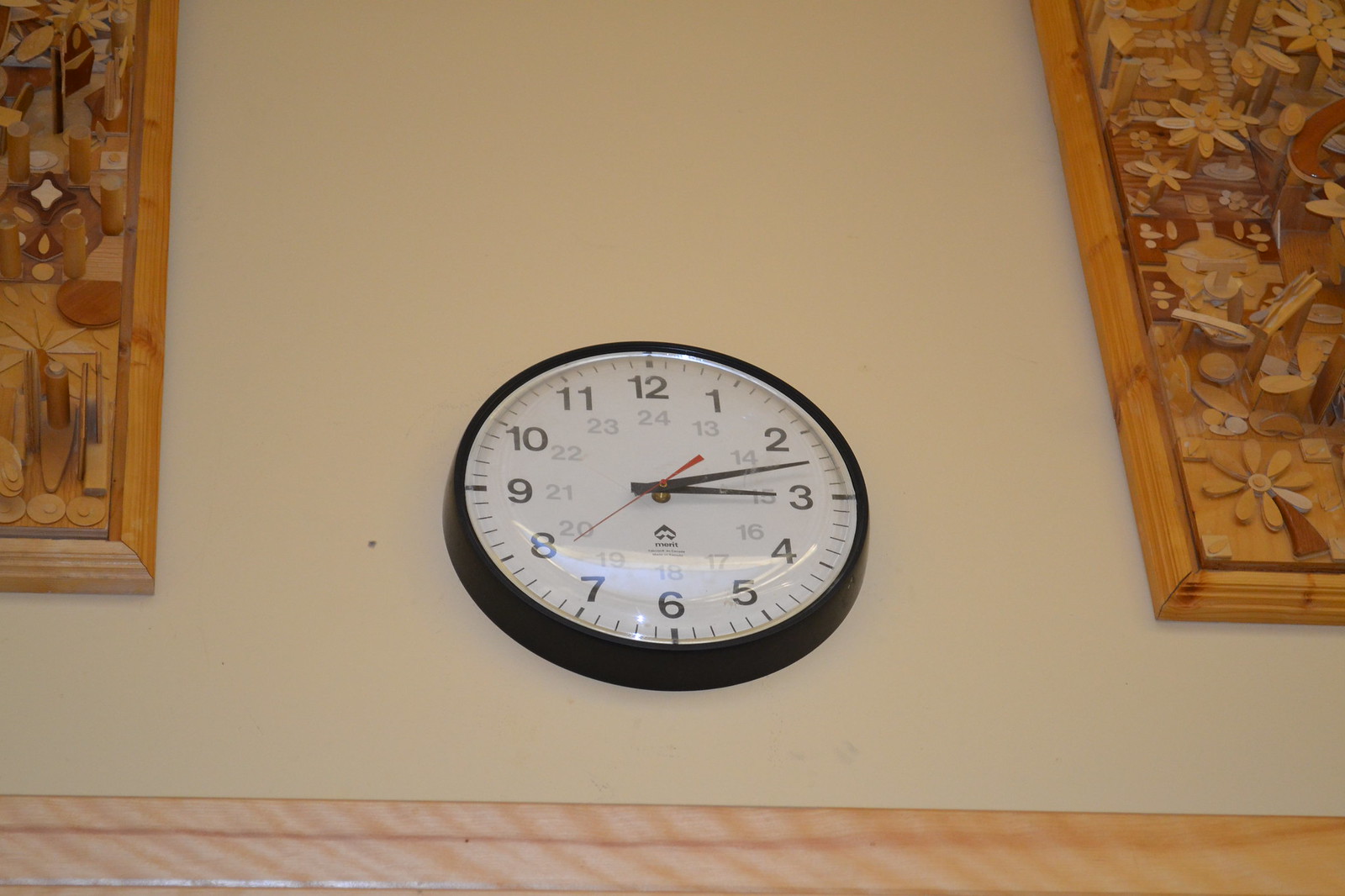The photograph captures a standard office-style wall clock mounted on a slightly yellowish wall. The clock features a thick black circular frame with a simple white face. Black numerals mark the hours with military time beneath them, and the time shows as 3:12. The clock’s minute and hour hands are black, while the second hand stands out in red. Flanking the clock on either side are two three-dimensional wooden artworks. These artworks consist of intricate designs with flowers made from small wooden pieces. The wall appears to be adorned with wooden wainscoting below the clock, suggesting it might be mounted either in a home or an office setting.